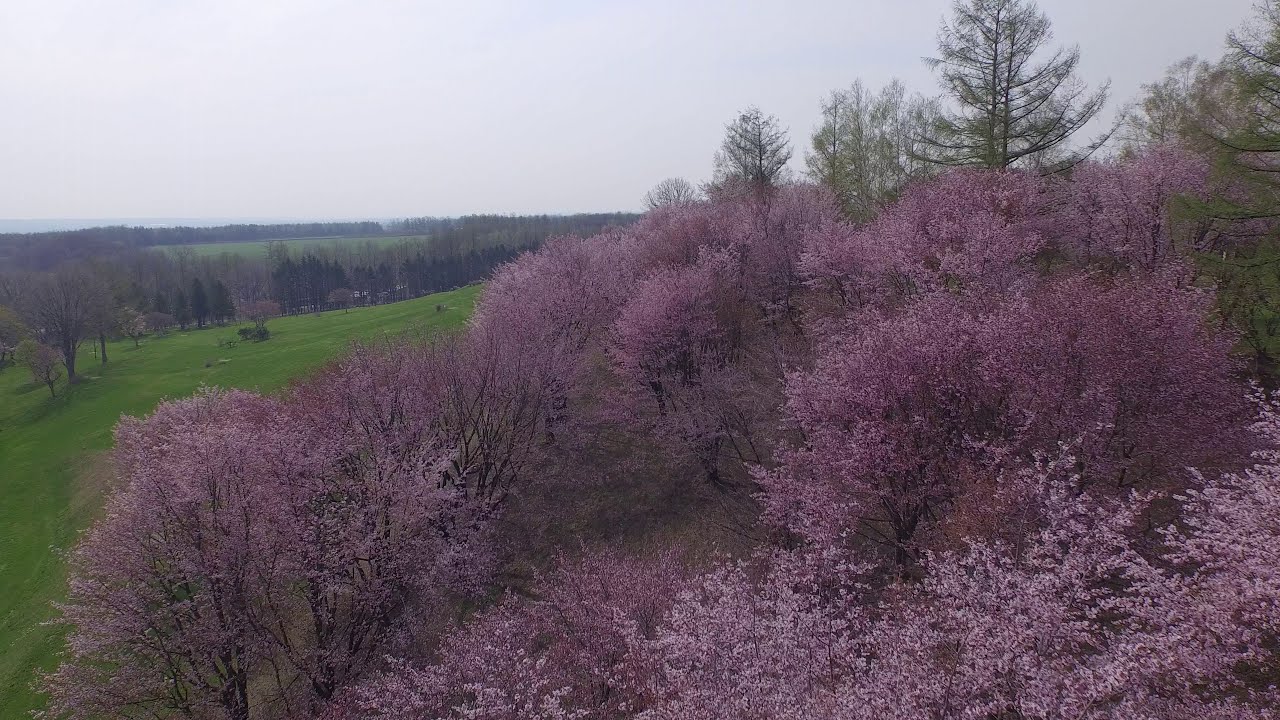This image captures a picturesque springtime landscape characterized by lush and vibrant scenery. In the bottom half of the image, there is a dense collection of trees adorned with beautiful lavender and pink blossoms, possibly cherry blossoms, set against a backdrop of green grass. In the foreground to the left, a hill covered in rich green grass adds to the verdant charm. The top right section hosts a grouping of traditional green and yellow trees, interspersed with some gray-tinged foliage that fades into the distance. The sky is overcast, painted in hues of white and light gray, contributing to the serene and somewhat melancholic atmosphere. The photograph appears to be someone’s capture of the countryside, possibly taken from an aerial perspective, showcasing the diverse and colorful palette of springtime flora against a tranquil sky.